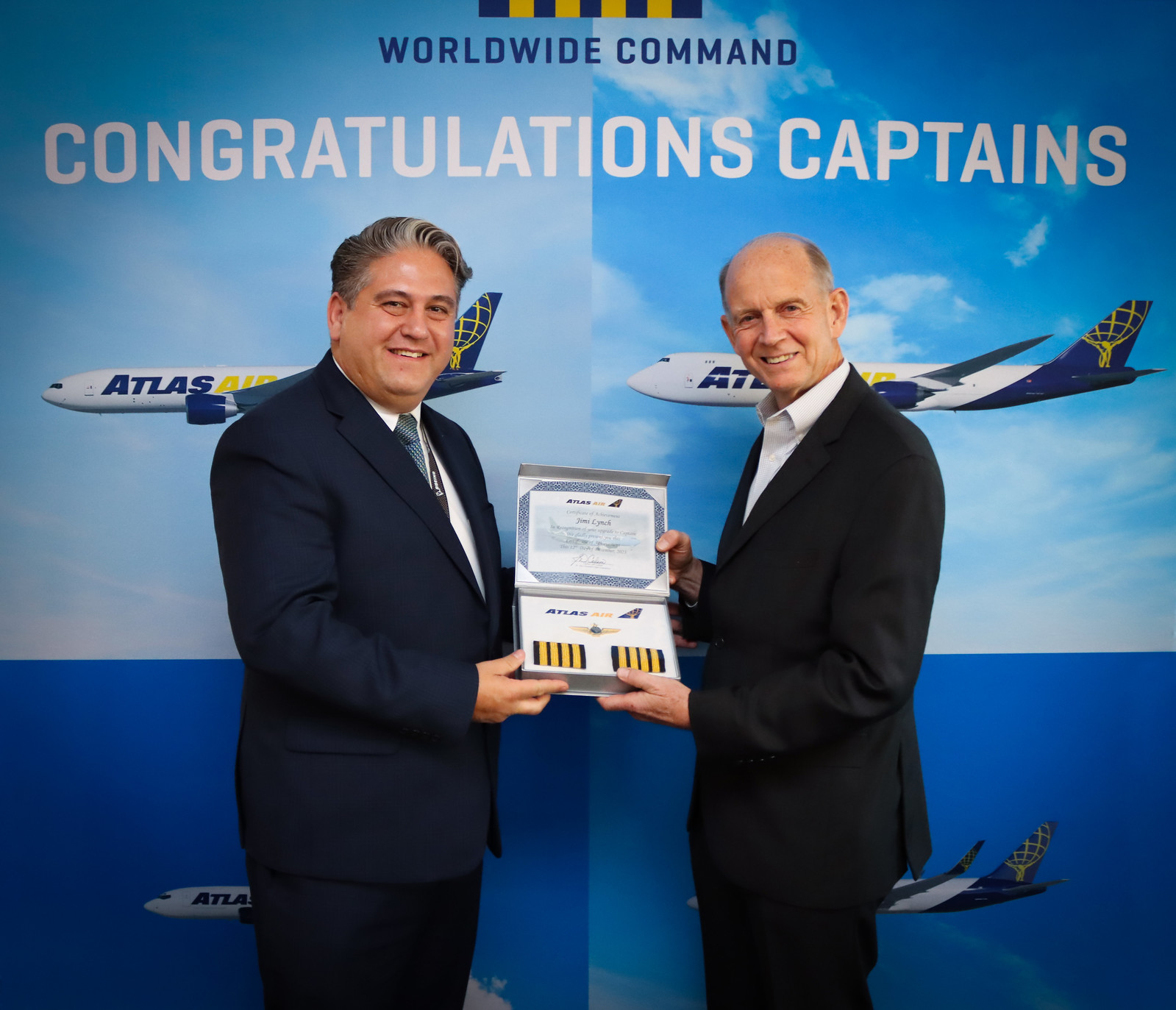The photograph depicts two middle-aged Caucasian men dressed in formal attire, celebrating a significant achievement. On the left, a man wearing navy blue dress pants, a matching business coat with a buttoned-up white collar shirt, and a blue tie adorned with white dots, stands with a black lanyard displaying white text around his neck. He holds a flip-open booklet containing a certificate and shoulder epaulettes – black and gold stripes indicative of a pilot's rank. Next to him, a man in black dress pants and a black button-up shirt with the top button undone holds the other side of the certificate. Both men are smiling at the camera, their bodies angled towards each other. Behind them is a display board featuring an airplane with text that reads "Worldwide Command. Congratulations, Captains." The airplane is marked with the "Atlas Air" logo. The image captures the significant moment of one man presenting a pilot’s certification and captain’s epaulettes to the other, likely celebrating a promotion to captain.